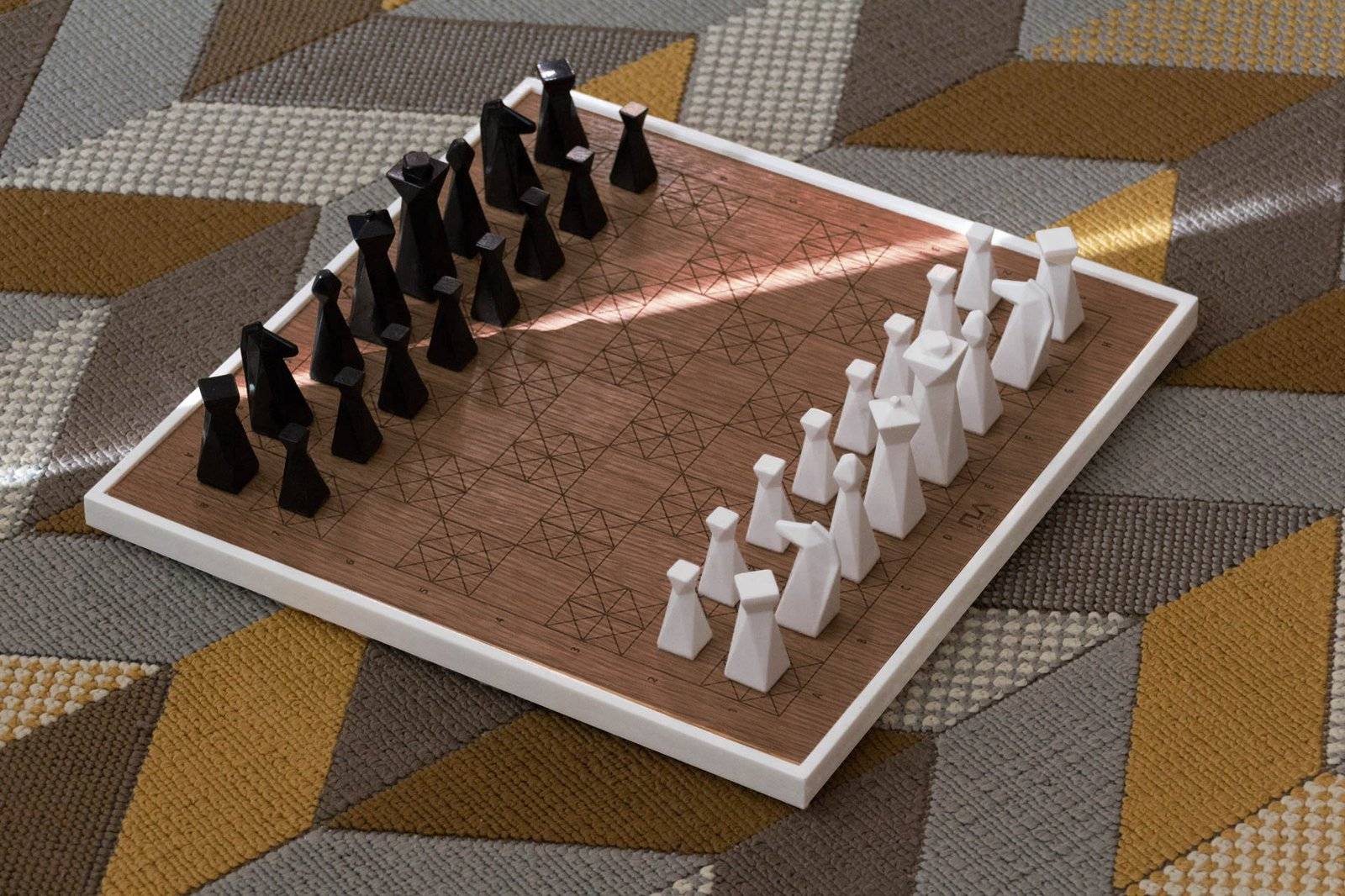The image depicts an indoor setting with a patterned carpet in shades of beige, gray, and brown, illuminated by a strip of sunlight. At the center is a distinctive chessboard, showcasing an intriguing design. The board features a white trim and a brown background with thin black lines forming squares, some containing smaller squares within them. The chess pieces are divided into black and white sides, positioned on opposite ends of the board. Notably, these pieces exhibit an unconventional, angular design, likely 3D-printed, with the smaller pieces having square fronts and triangular pyramid-shaped bases, while the taller ones showcase unique, identifiable tops. The board and pieces rest on a wooden surface, blending traditional elements with modern design in a homely environment.